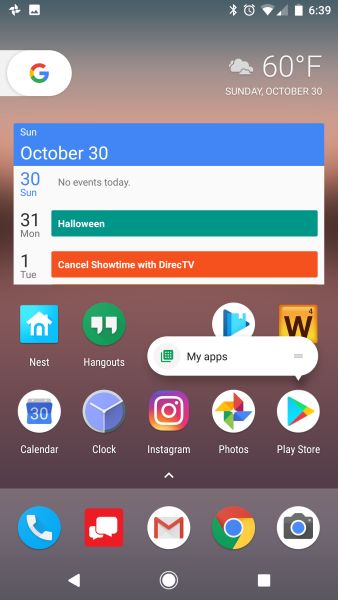This image captures a detailed view of a smartphone screen showcasing various elements. The background transitions seamlessly from gray at the top, blending through light tan to dark brown, before reverting to gray at the bottom. In the upper left corner, there is a colorful Google Photos pinwheel icon positioned next to a picture icon. On the upper right, white icons display the current time, Bluetooth, alarm, Wi-Fi signal strength, and battery level.

Below this status information, on the right-hand side, there is a weather widget showing a white cloud icon and a temperature of 60°F with the date Sunday, October 20th. On the left-hand side of the screen, there's a white Google Assistant search bar with the multicolored Google "G" logo.

Dominating the middle of the screen is the calendar window, topped by a blue banner with the date reiterated as Sunday, October 30th. The calendar notes no events for the 30th, but highlights a green bar for Halloween on the 31st and a red bar for "Cancel Showtime with DirecTV" on the 1st.

The lower portion of the screen organizes various application icons into rows. The first row includes apps for Nest, Hangouts, Google Play, and Words with Friends. The second row features Calendar, Clock, Instagram, Photos, and Play Store apps. Along the bottom row, essential functions are represented with icons for Phone, Text Messaging, Gmail, Chrome, and Camera.